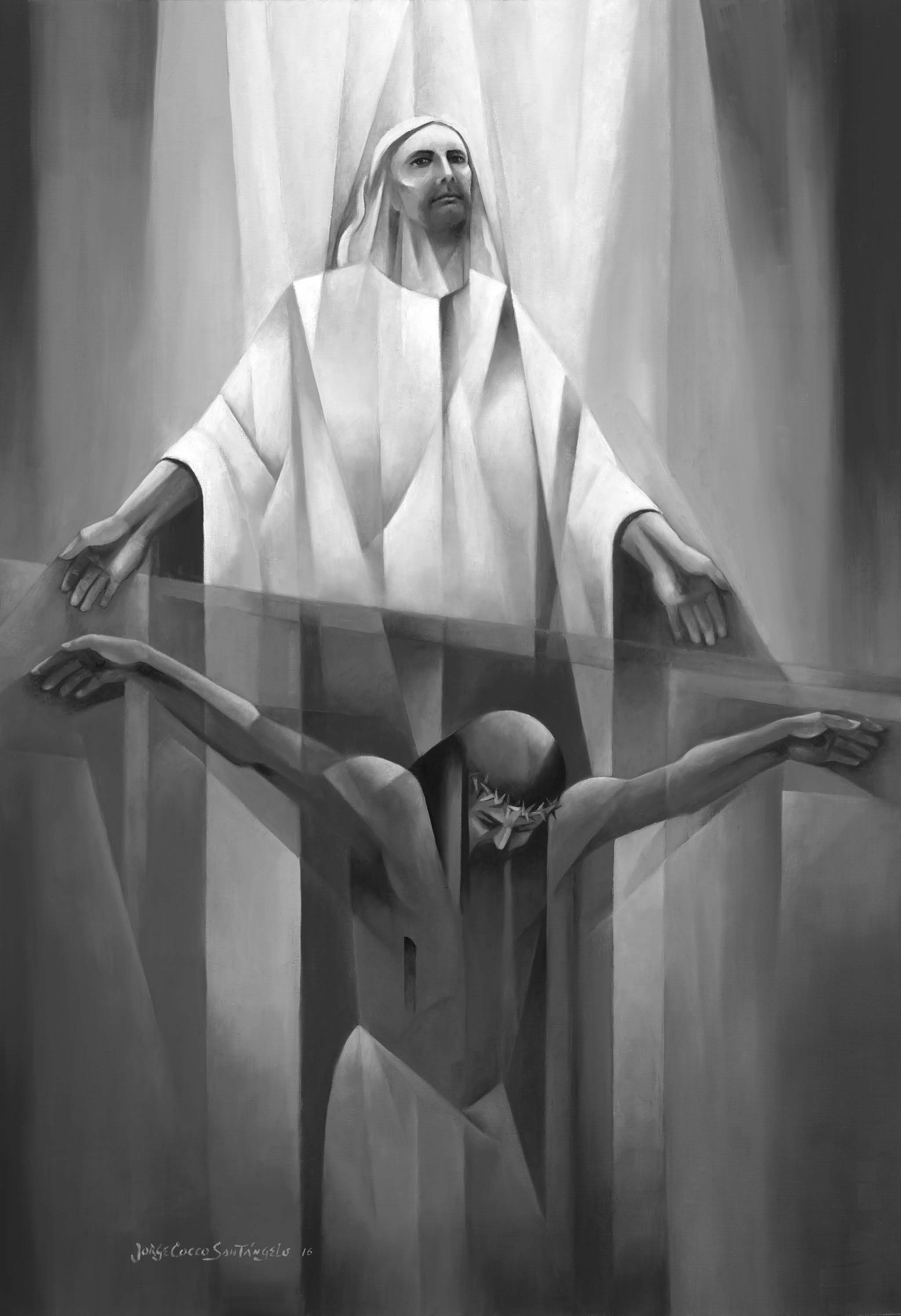This black and white drawing, starkly composed of straight lines, features a compelling depiction of Christ's crucifixion. At the bottom half of the image, Christ is shown with his arms held up against the cross, his head tilting down under a crown of thorns. His skin is rendered in gray tones with pronounced shadows, and a white cloth is modestly wrapped around his waist. A small, barely legible signature appears in the bottom left corner.

Above Christ, on the top half of the drawing, stands another man. His upper torso and head are depicted, with his arms reaching down towards Christ's hands. He wears a white cloth apron draped around his body and on his head, and his gaze is directed upwards. His mouth and chin are darkly shadowed. The background transitions from a white space behind the upper figure to a darker gray outside, suggestive of draped curtains. The entire composition is rich in tonal contrasts and meticulously detailed, capturing both the solemnity and the tension of the scene.